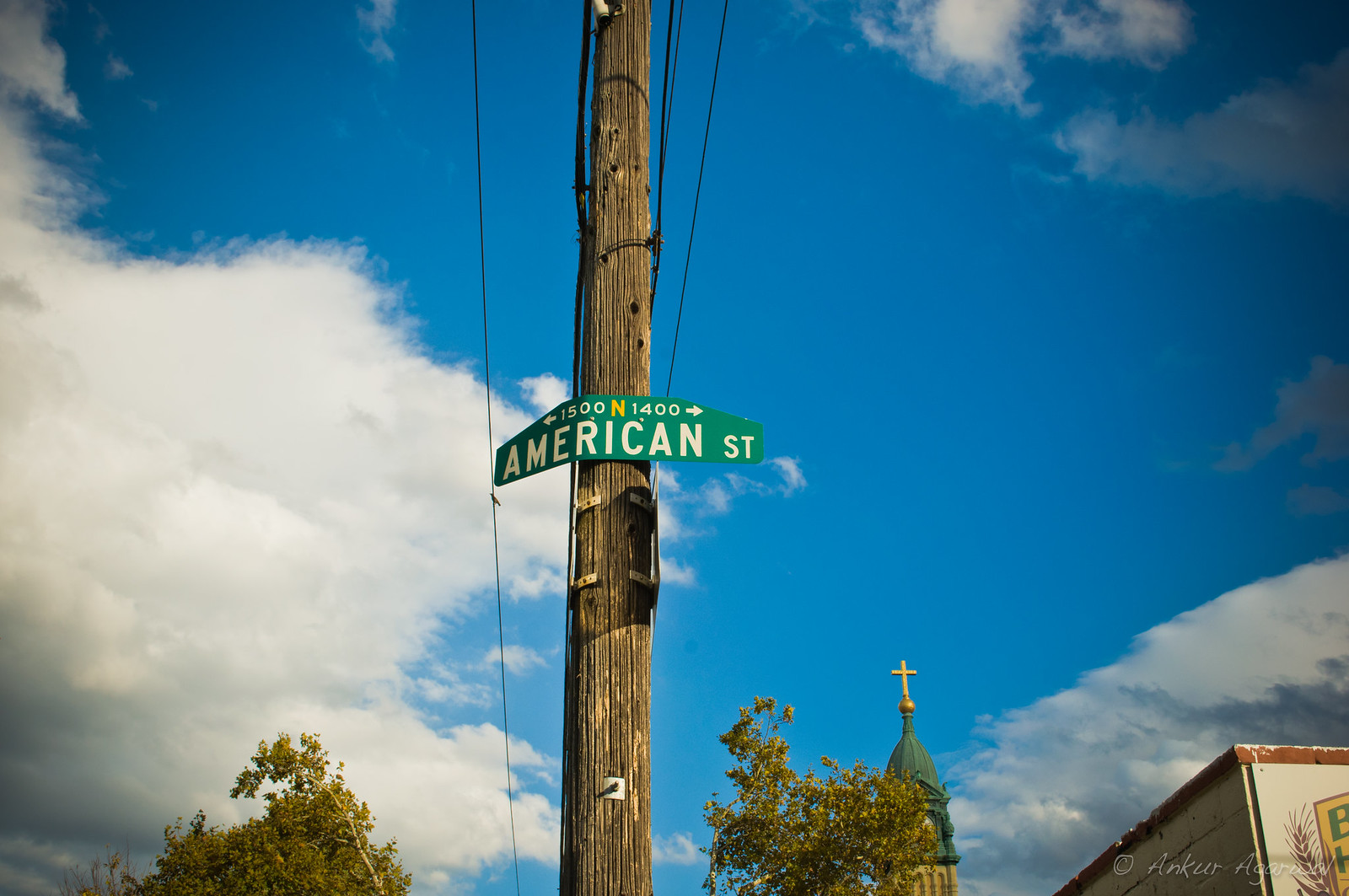In this realistic outdoor photograph taken from a lower vantage point looking upward, the bright blue sky is scattered with white, fluffy clouds. Dominating the lower portion of the image are the tops of two trees, their green foliage contrasting with the brilliant sky. A weathered, wooden utility pole stands prominently in the center, extending from the bottom to the top of the frame. Attached to the pole is a slightly bent, green street sign that reads "American Street." The sign includes directional arrows pointing left and right, marked with "1500 N" in yellow and "1400" below it in white. Electrical wires extend from the pole into the distance, adding depth to the scene.

To the right, the photograph captures the upper tower of a church. The church's steeple is circular with a green roof that supports a gold ball topped by a gold cross, gleaming against the sky. A cream ivory building with a weathered red border is visible behind the utility pole, contributing to the urban setting. Adding a final touch of realism, a small watermark is noticeable in the lower right corner, reading "A-N-K-U-R" followed by "A-G."